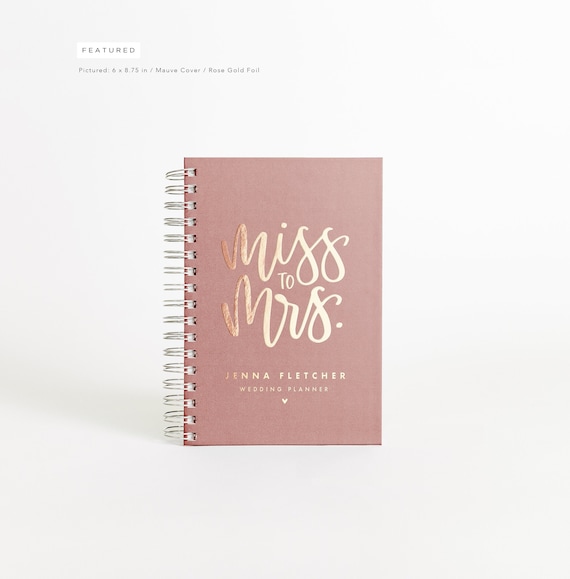The image is a professionally rendered photograph of a 6 by 8.75 inch spiral notebook, suitable for sale, shot against a very light gray to white background. At the top of the image, there is a white rectangular box with the word "featured" in dark gray print, followed by the specifications "6 by 8.75 inch / mauve cover / rose gold foil." 

The notebook itself has large white spirals on the left side and a light pink (mauve) cover. In the center of the cover, elegant cursive rose gold foil lettering prominently displays the phrase "Miss to Mrs." Below this, in smaller rose gold print, the name "Jenna Fletcher" is inscribed, followed by the title "wedding planner" in even smaller print. Beneath this final line, a delicate gold heart symbol completes the design. This image appears to be a promotional piece likely featured on Jenna Fletcher's website, either as a product for sale or as part of her advertisement for wedding planning services.